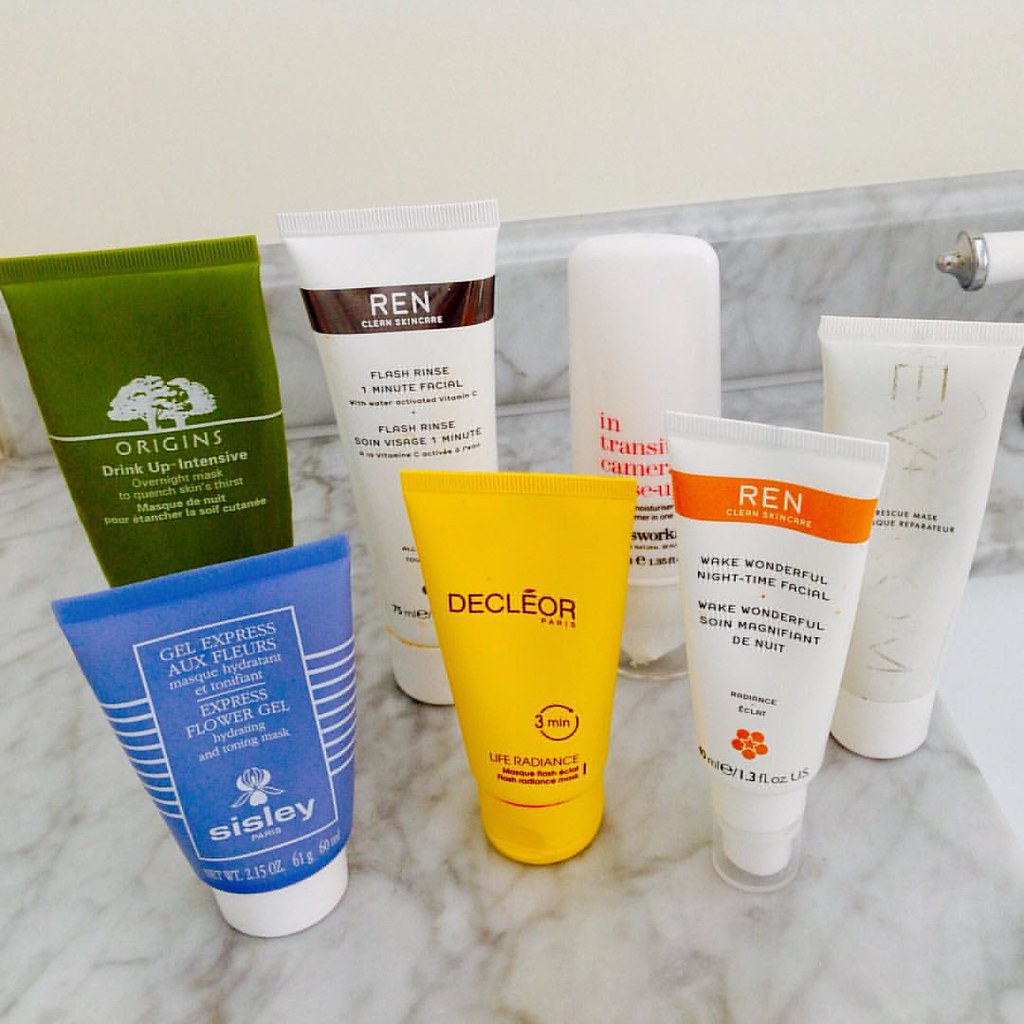A detailed photograph showcasing a bathroom vanity with a pristine white marble countertop adorned with an assortment of beauty products. The forefront of the image highlights a sky-blue squeeze bottle labeled Sisley, featuring the "Express Flower Gel Hydrating and Toning Mask." Beside it, a bright yellow squeeze bottle from Decléor Paris captures attention, with its distinctive logo and "Life Radiance" inscription. A white squeeze bottle of "Wake Wonderful Night-Time Facial" from Ren Clean Skincare stands nearby, complemented by another Ren product, the "Flash Rinse 1 Minute Facial," distinguished by its white bottle with a brown banner. Tucked behind the Sisley product, a green Origins bottle labeled "Drink Up Intensive Overnight Mask" peeks out. Additionally, one can spot another white squeeze bottle with indistinct labeling due to slight blurring. Lastly, an intriguing non-squeeze bottle, partially obscured, bears the somewhat obscured text "In Transit Camera," adding an element of mystery to this elegant and neatly arranged beauty ensemble.